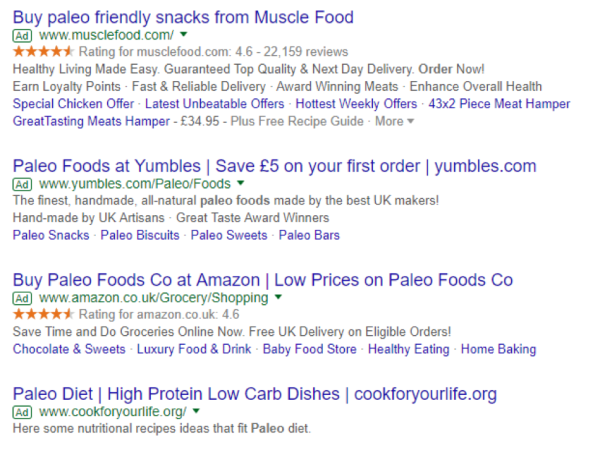In this image, a Google search results page is displayed, with all visible entries being advertisements. The first entry promotes "Paleo-Friendly Snacks" from MuscleFood, featuring a 4.6-star rating based on 22,159 reviews. The ad highlights benefits such as "Healthy living made easy," "Guaranteed top quality," "Next day delivery," "Order now and earn loyalty points," "Fast and reliable delivery," "Award-winning meats," "Enhanced overall health," and special offers like a "43-piece meat hamper" and "Special chicken offer."

The second result is an advertisement for "Paleo Foods at Yumbo's," offering a £5 discount on the first order. The URL is www.yumbos.com/paleo/food.

The third ad promotes purchasing "Paleo Foods at Amazon," emphasizing low prices. The corresponding URL is www.amazon.co.uk/grocery/shopping.